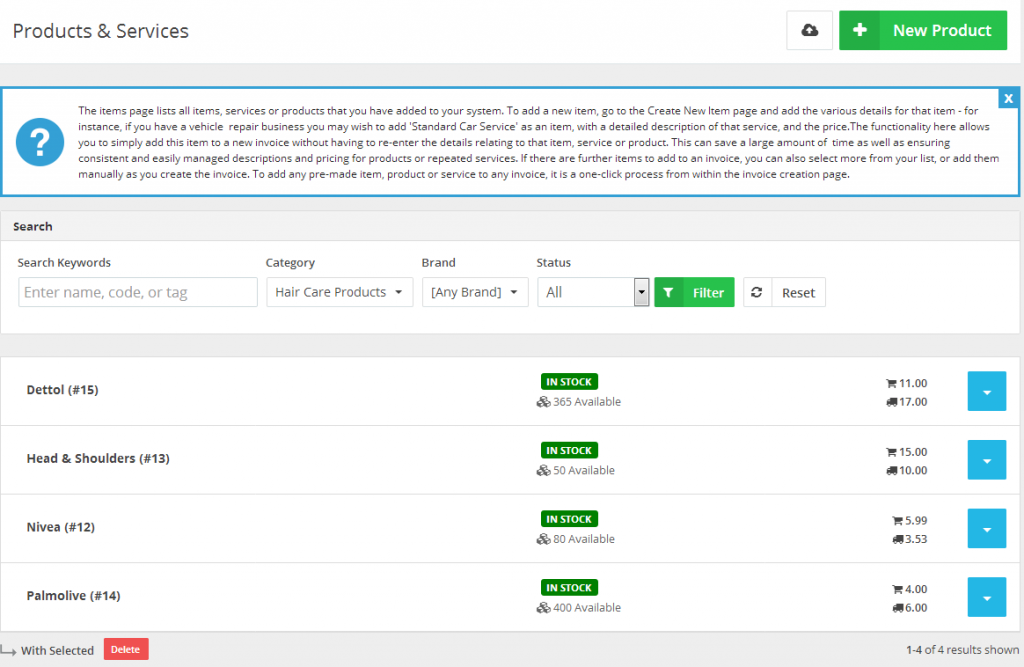The image depicts an online store's checkout cart interface, designed with a wider-than-tall format and a predominantly white background. At the top of the screen, on a white banner, the words "Products and Services" appear in the upper left-hand corner. Beside this text, there is a green box containing a white arrow and the phrase "New Product" also written in white. Below this section, a large box with a blue border is visible.

This large box contains a section labeled “Items” that lists all added products or services and provides a five-line set of instructions on how to utilize this page effectively. Below the instructions, there are several functional elements for user interaction. These elements include a search function, a search box, a category drop-down menu, a brand drop-down menu, a status drop-down menu, a green "Filter" button, and a white "Reset" button.

The shopping cart currently contains four items, each marked as in stock with green rectangles indicating their availability. The items and their respective statuses are as follows:
- **Dettol**: Priced at 11 units for in-store pickup and 17 units for delivery.
- **Head & Shoulders**: Price details not specified.
- **Nivea**: Price details not specified.
- **Palmolive**: Price details not specified.

All listed items include the options for in-store pickup or delivery, each with either a specific price or status indicator.